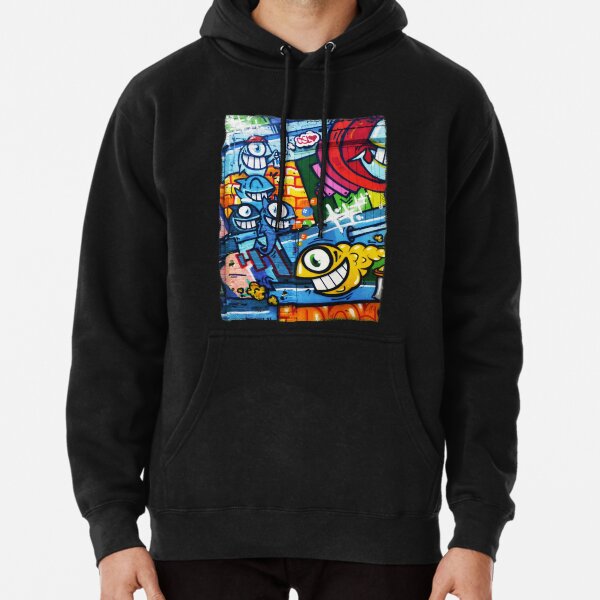This photograph features a young male model, whose head is out of frame, showcasing a black hooded sweatshirt against a plain white background. The hood is down, revealing two drawstrings hanging from the neckline. The main focal point of the sweatshirt is a vibrant, colorful square graphic centered on the chest. This graphic includes a collection of cartoonish creatures resembling one-eyed, large-toothed sharks or monster-like fish. These characters are depicted in a palette that spans red, lavender, green, blue, orange, and gold, evoking a street art or animated video game aesthetic. The vivid scene includes elements that suggest a road, brick wall, and green area, adding dynamic interest to the otherwise dark garment.